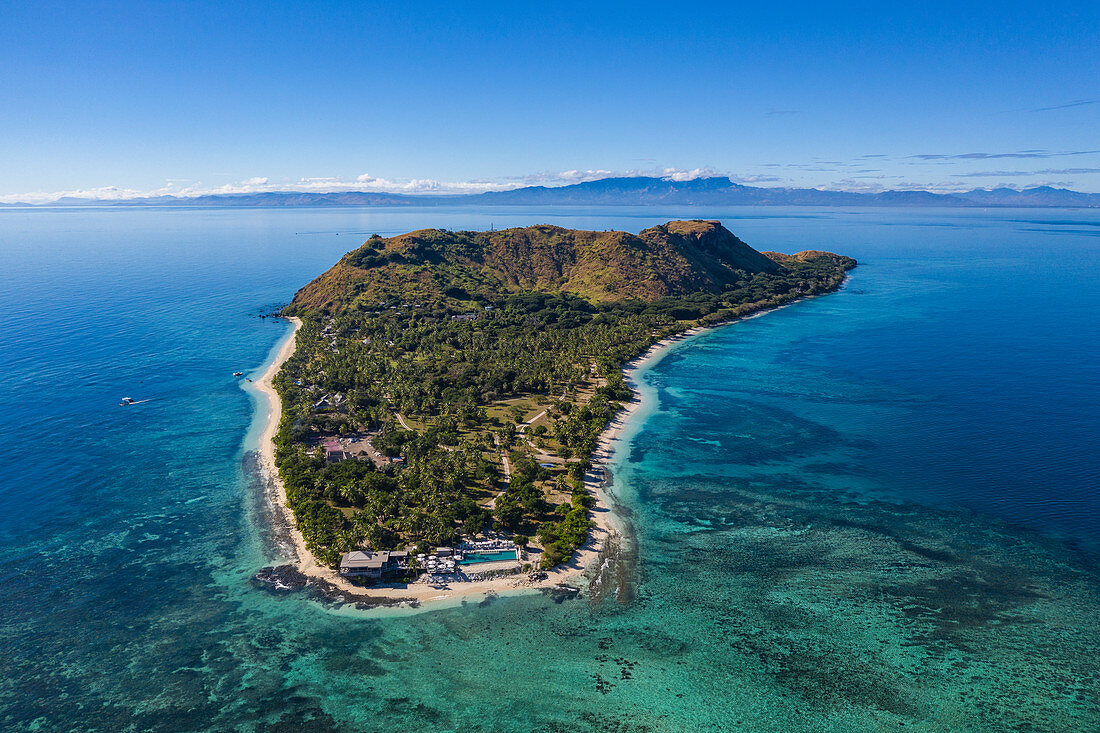An aerial view of a stunning tropical island set in a vibrant blue ocean. The island, shaped like a crescent or a curved oval, occupies the center of the image and is covered in lush greenery with dense trees. At the rear of the island, mountainous terrain creates a dramatic backdrop, potentially harboring a volcanic structure. The fertile green expanse transitions into pristine white sandy beaches that outline most of the island’s perimeter. Visible from above, there are a few small buildings and a swimming pool near the front shore, along with roads that wind through the island connecting the eastern and western shores, where additional buildings and parking lots are located. Boats gently float in the shallow, aqua-colored waters on the west coast, contrasting with the deeper sapphire blue waters further out. Distant mountains and clouds adorn the horizon, blending into a beautiful blue sky. The scene encapsulates the stunning interplay of varied blues of the ocean and sky with the greens and whites of the island, making it a breathtaking and picturesque landscape.